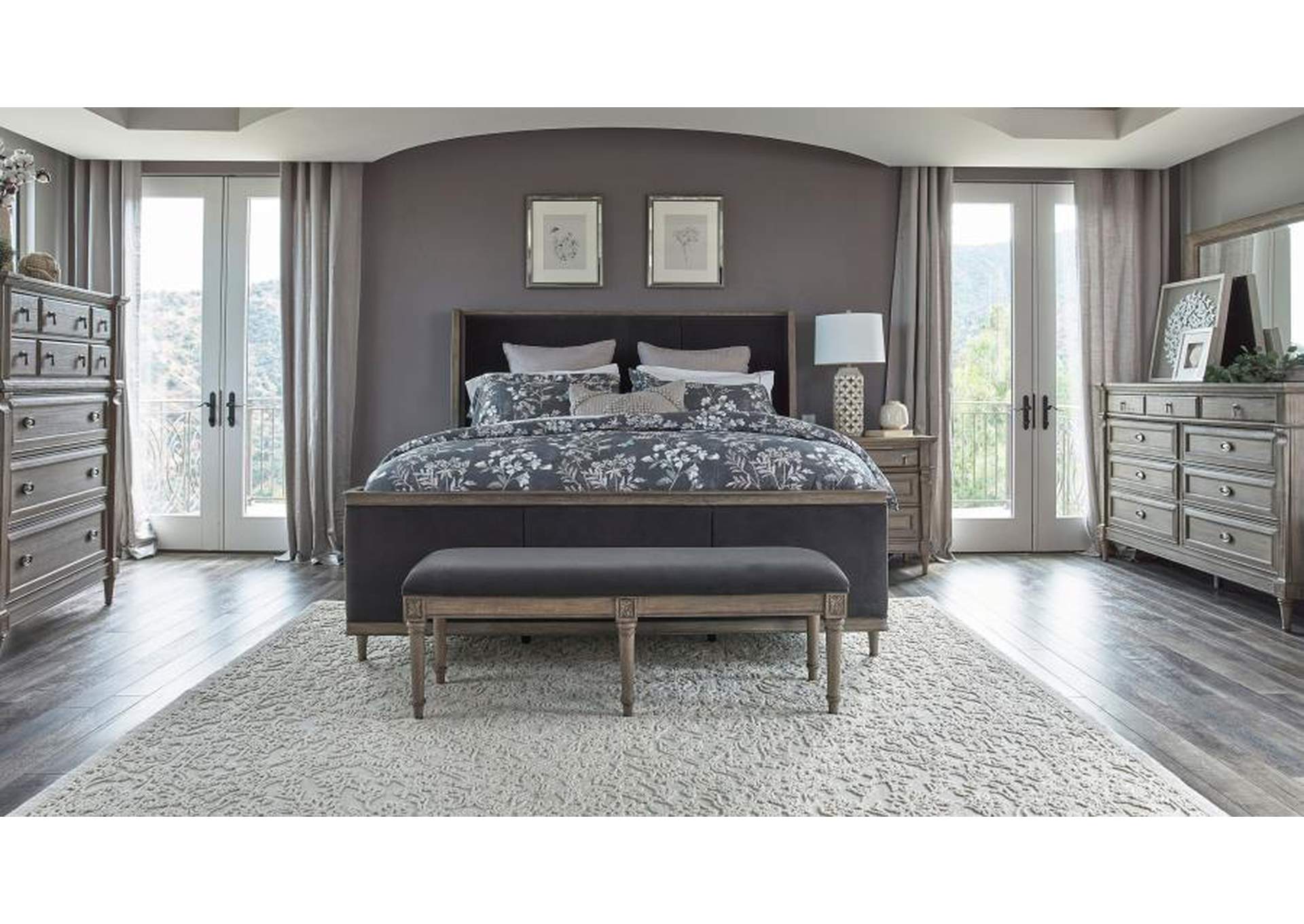The photo captures a bright, daytime scene inside a well-appointed bedroom, likely in an apartment. At the center of the room is a large bed with a dark gray rectangular headboard, adorned with multiple throw pillows in various shades of white and gray. A bedspread adorned with a white flower print covers the bed, which is complemented by matching throws. At the foot of the bed sits a gray settee with six legs.

The floor is covered in light gray-colored wood planks, and beneath the bed and bench lies a large, square-shaped light gray rug. Directly above the bed are two framed photographs, adding a touch of elegance to the space.

Flanking the bed on both sides are nightstands, each topped with a lamp. Additionally, light gray dressers are positioned on either side of the room. At the far end of the bedroom, French doors with clear glass panes and sheer curtains stand open, revealing a view of the outdoors and allowing ample daylight to stream into the room. Subtle touches like the well-arranged clothing shelves in the corners complete the cozy and welcoming atmosphere of the bedroom.